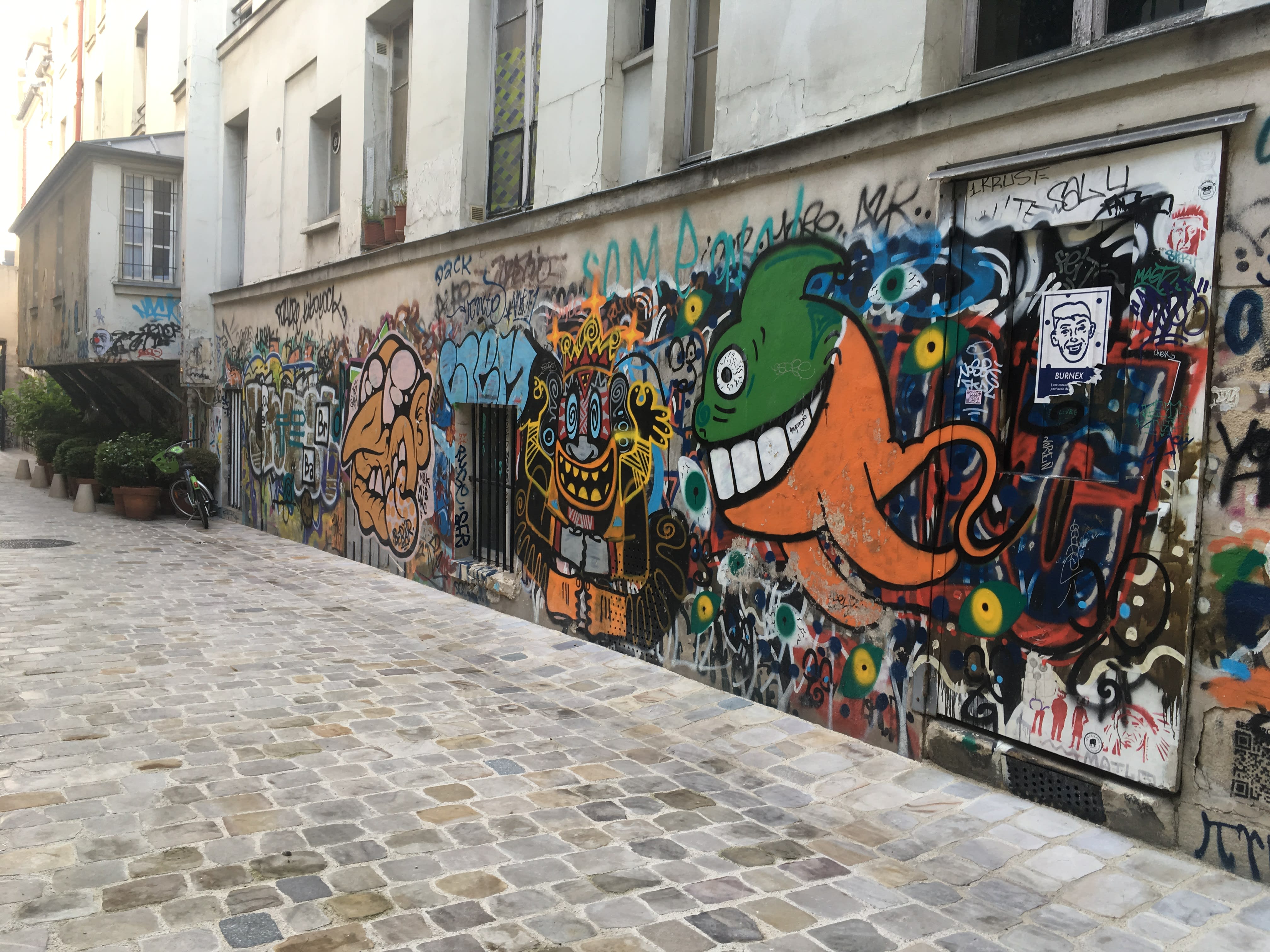The image depicts a vibrant urban street scene centered around a residential apartment building with its lower 10 feet covered in professional, multicolored graffiti. This artistic wall features a variety of characters, including a large smiling fish, an intricate voodoo monster, an exaggerated face with a dangling tongue and glasses, all intertwined with graffiti writing and colorful elements like green and yellow eyeballs. Above the graffiti, the off-white building has several windows, some of which have bars. To make the scene more dynamic, a hangover structure extends from the left side of the building, supported by wooden pillars, sheltering a collection of potted plants and a small bicycle below it. The street in front consists of cobblestones in a medley of grays, tans, and beiges, adding texture and color to the urban setting.